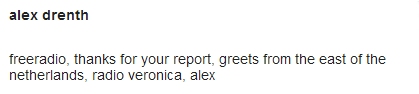The image features a solid white background with black, sans serif text. In the top left corner, in bold lowercase letters, it reads "Alex Drenthe, A-L-E-X D-R-E-N-T-H." Beneath this, in non-bolded, lowercase text of the same font style, it says: "free radio, thanks for your report, greets from the east of the Netherlands, radio Veronica, Alex." The rest of the image is simply blank with no other graphical elements or images, resembling a typed message or a digital note.